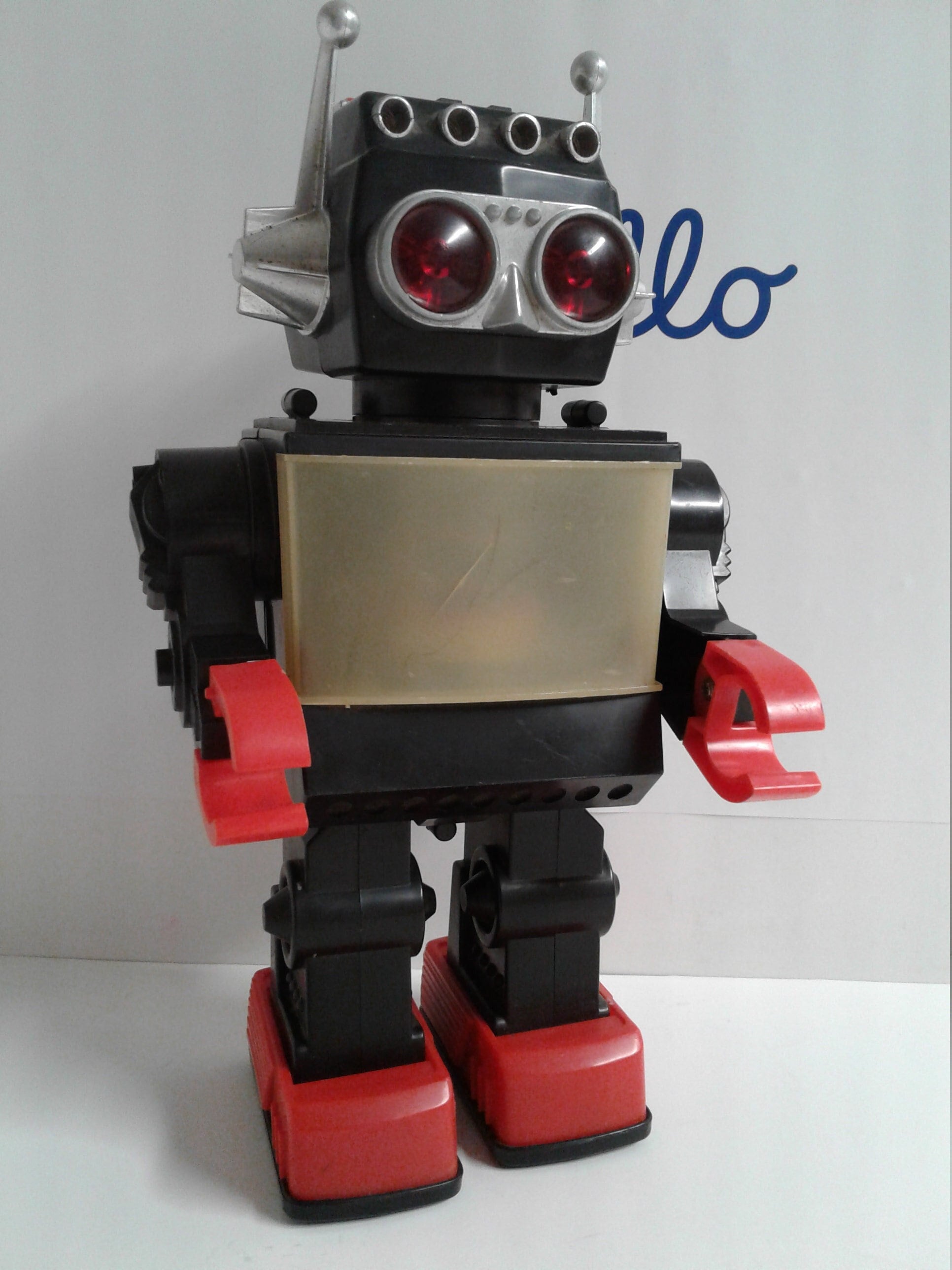The image features a retro-styled robot toy that appears primarily black, with elements in red, silver, and bronze. The robot is constructed from what seems to be hard plastic. Its most striking features include red hands and feet that resemble those of a Lego character. The robot’s red eyes look like translucent gemstones set within silver, and it has two silver antennas with small balls on the ends. The chest plate is cream-colored, adding a bit of contrast to its black body. The robot's arms are bent at the elbows, and it has articulated knees, suggesting it might be a wind-up toy, although the wind-up mechanism isn't visible. The background includes a white floor and a gray wall with partially obscured blue text that likely reads "hello."